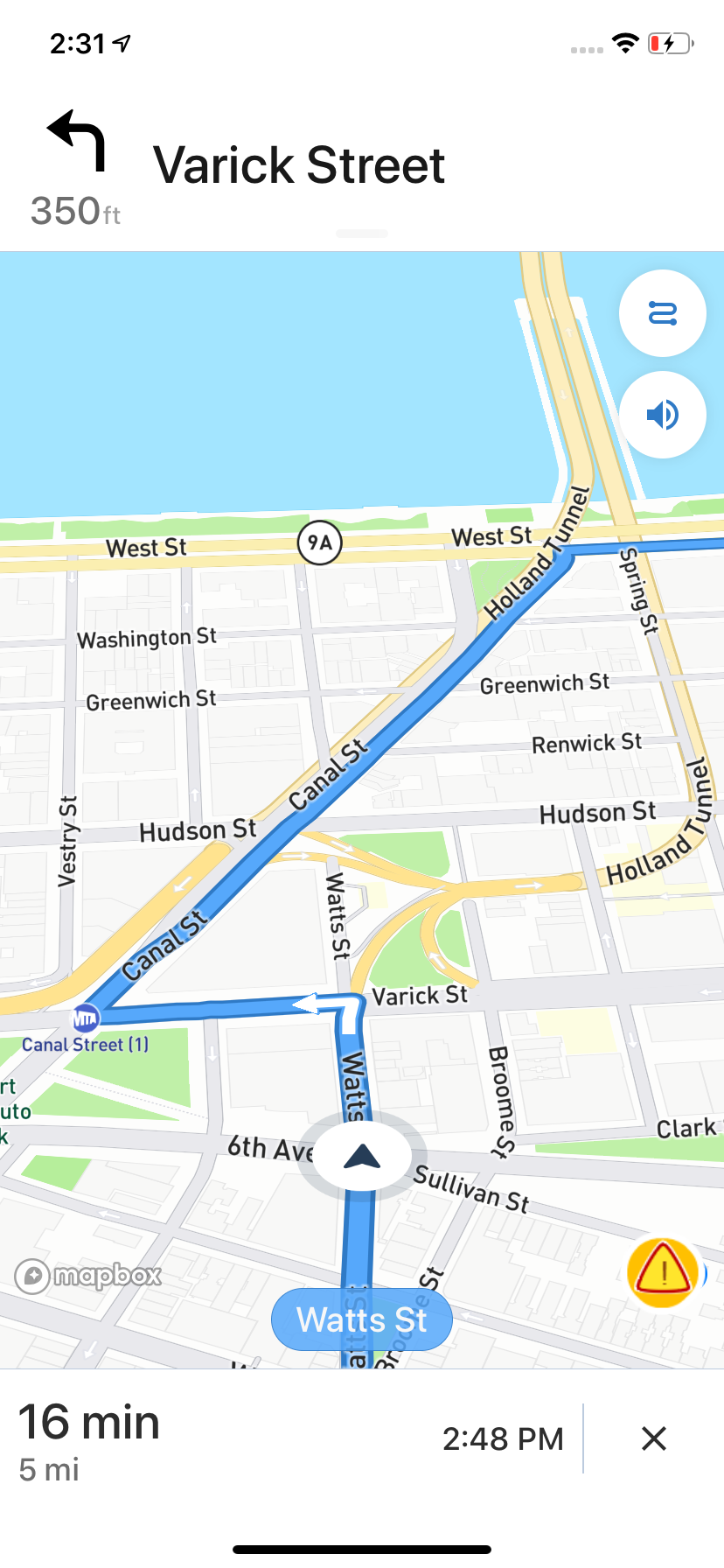Screenshot of a GPS Navigation App

This image is a screenshot captured from a cell phone, displaying a navigation screen of an unspecified GPS app. The top section of the screen includes standard smartphone indicators such as the time, Wi-Fi signal, and battery level. Dominating the image is a map interface, reflecting a routed navigation path.

At the very top of the map, there's an instruction for the next step in the journey. It directs the user to make a left-hand turn in 350 feet onto Verrick Street. This instruction is represented by a leftward arrow symbol, without accompanying text. 

Below this directive lies the navigation map itself, which is rendered in a simplified, drawn format rather than a satellite view. The map details a path beginning at Watts Street, continuing to Verrick Street, followed by Canal Street. The final destination is not visible in this screenshot. The current location is highlighted as Watts Street.

Beneath the map, essential journey details are provided. The estimated travel time to the destination is 16 minutes, covering a distance of 5 miles, with an expected arrival time of 2:48 PM. An 'X' button is available in this section, offering an option to exit the navigation.